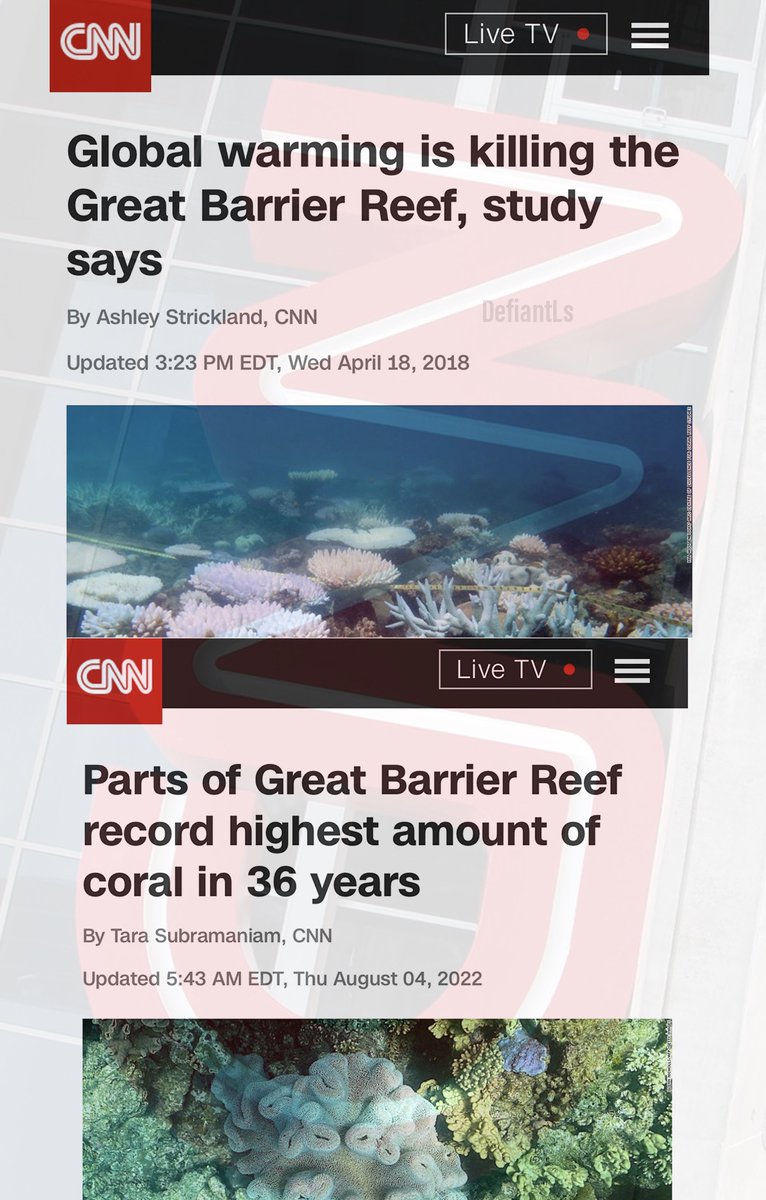A long-format screenshot, likely captured from a mobile device, showcasing the CNN website. The background appears as a white overlay, potentially superimposed on an image of the CNN building. At the top of the screen, the iconic CNN logo is displayed in red, accompanied by a black bar with a 'Live TV' button marked by a red dot, and a three-horizontal-line menu icon.

Below this header is black text reading: "Global warming is killing the Great Barrier Reef, study says," authored by Ashley Strickland, CNN, with an update timestamp of 3:23 PM EDT, Wednesday, April 18th, 2018. This is followed by an image depicting the Great Barrier Reef, watermarked with "Defiant LS".

Further down, the CNN logo reappears with the same black bar featuring the 'Live TV' button and menu icon. Underneath, new text reads: "Parts of Great Barrier Reef record highest amount of coral in 36 years," written by Tara Subramaniam, CNN, updated at 5:43 AM EDT, Thursday, August 4th, 2022. Another image of coral is shown below this text. The screenshot seems to highlight different stories concerning the Great Barrier Reef, spanning over several years.